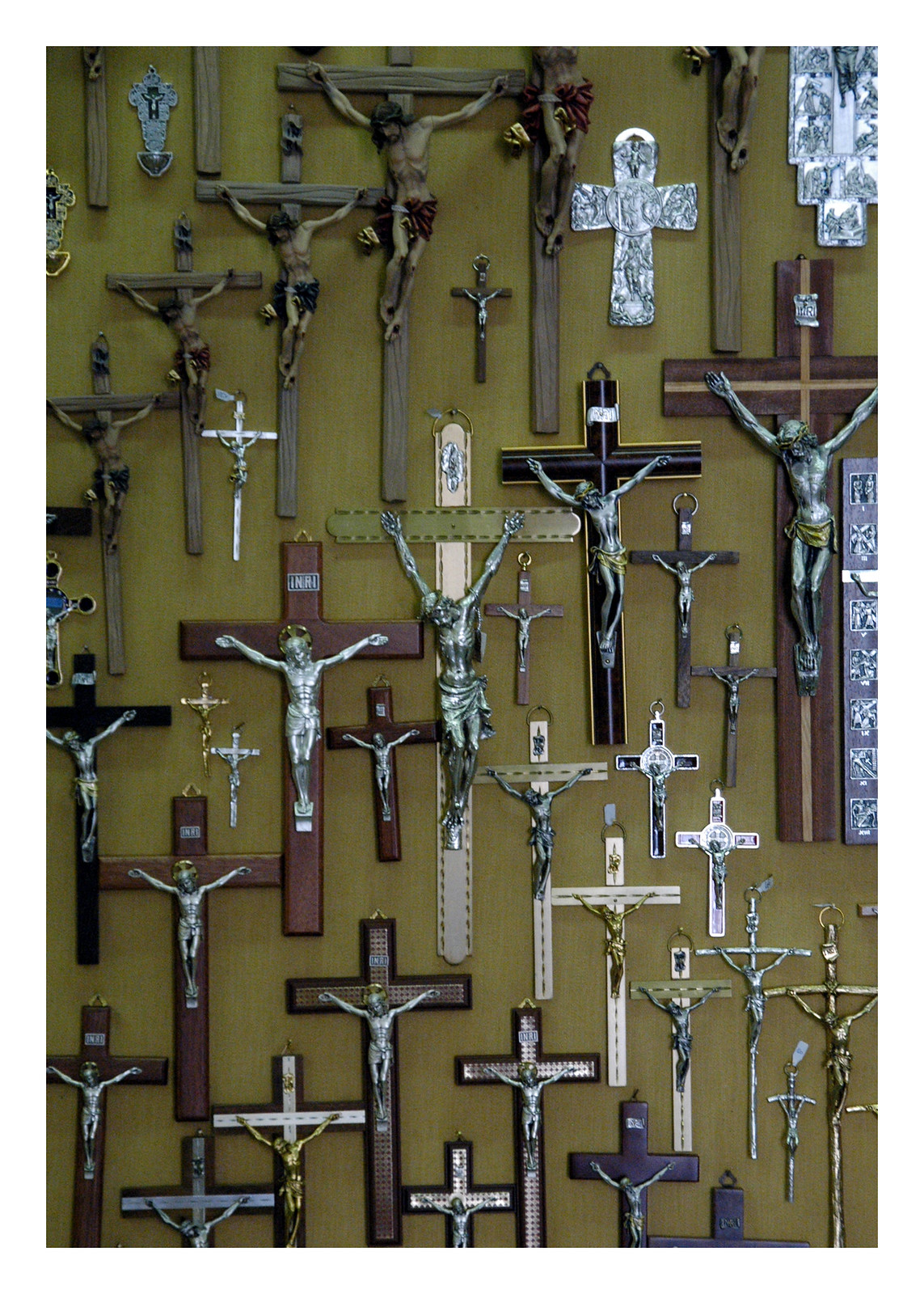The photograph displays a diverse collection of crucifixes meticulously arranged on a yellowish-green wall, potentially indicating they might be for sale given the variety. Dominating the center is a distinctive gold crucifix, adorned with small dots, that resembles the form of a sword or a thin belt. Surrounding it are numerous other crucifixes of varying shapes, sizes, and materials, including different types of wood, gold, silver, pewter, and bronze. The depiction of Jesus Christ is present on most crosses, detailed in various colors such as silver with gold attire, or brown with dark brown hair. Some crosses, particularly toward the top right, lack the figure of Jesus and appear more elegant, possibly vintage. Unique among them is an Egyptian cross, standing out due to its distinct design. Many crosses are intricately decorated, featuring carved wooden channels or pewter embellishments, showcasing both the craftsmanship and the spiritual symbolism of these religious artifacts.